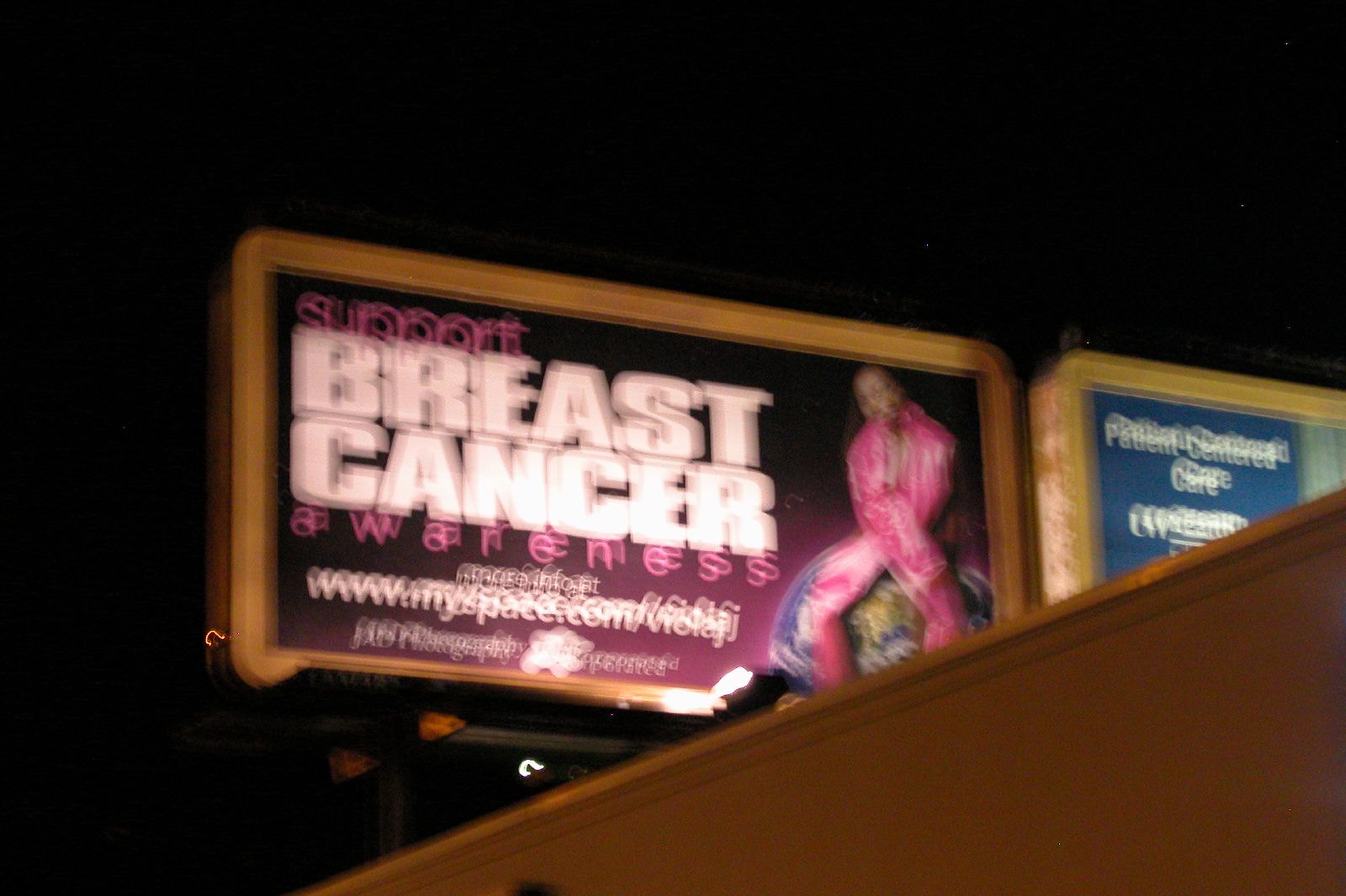Captured during the night, this very blurry photograph features two billboards against a pitch-black sky. The primary billboard showcases a powerful message supporting breast cancer awareness, prominently displayed in large white letters with pink highlights. A figure, dressed in pink, is visible on the far right side of this billboard, though the text below them is unreadable due to the blur. Adjacent to this, another billboard with a brown border is partially visible. It includes a blue box with white lettering, rendered illegible by the motion blur. In the bottom right corner, a brown ledge obscures part of the image, adding to the frame's chaotic yet poignant composition.